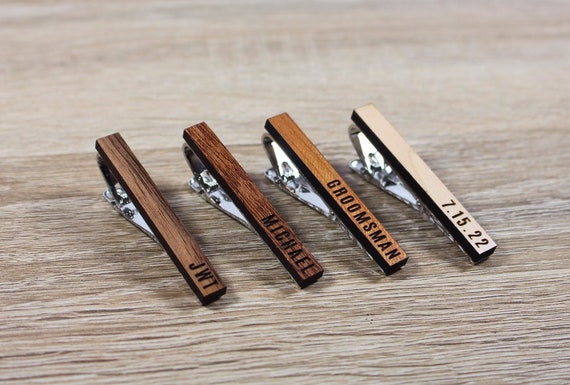This image displays four distinct wooden tie clips arranged neatly on a lightly hued, grayish wooden table. Each tie clip has its own unique wood grain and color, positioned from right to left. The first clip, almost white with a wood grain texture, is engraved with the date "7-15-22." The second clip, resembling light pine wood, features the word "Groomsman." The third clip, with a rich cherry or oak-like appearance, is engraved with the name "Michael." The fourth clip, colored in a grayish-brownish wood, bears the initials "JWT." The metal clips on the back of each wooden piece are silver, designed to easily attach to a tie. The engravings appear indented into the surface of the wood, adding a tactile element to their aesthetic. The table's wood appears unfinished, contributing a subtle, rustic charm to the composition of the tie clips.